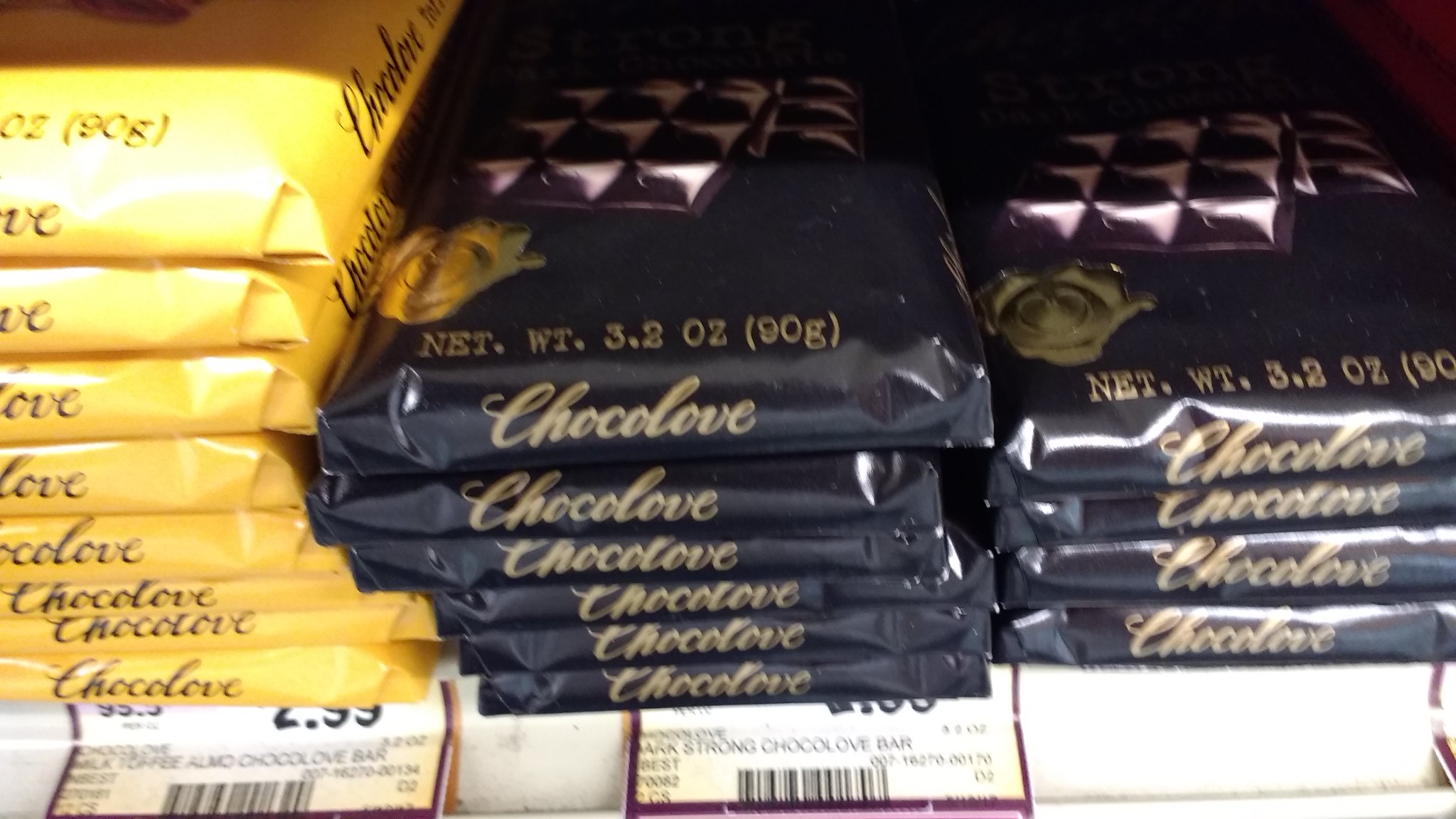The image depicts a shelf stocked with various chocolate bars. On the right-hand side, there are eight large Choco Love bars wrapped in yellow packaging. The yellow wrappers feature the text "Choco Love" prominently on the side, each weighing 90 grams. A sign beneath this section indicates that these yellow-wrapped chocolate bars are priced at $2.99 each. 

To their left, there are two columns of Choco Love bars in black wrappers. The black packaging also states "Choco Love" in gold lettering, with an image of chocolate displayed on the top. Each of these bars also weighs 90 grams (3.2 ounces). The price for these bars is not clearly visible due to the positioning of the first column, which consists of six bars, while the column on the far left contains four bars.